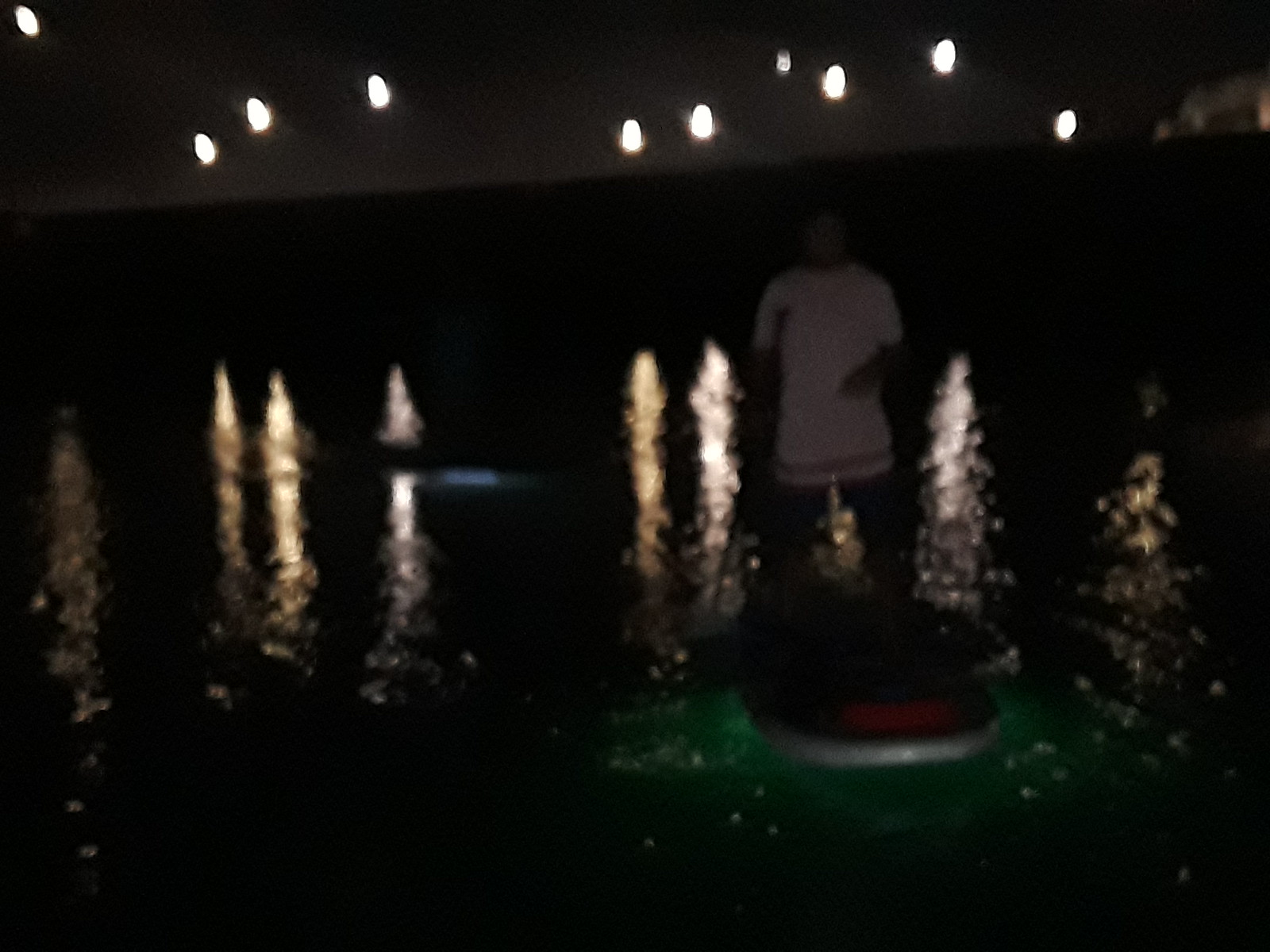A captivating night scene features a woman standing on a boat, draped in an oversized, white, short-sleeve shirt that resembles a gown, paired with blue jeans or possibly blue jean shorts. She holds a paddle in one hand, while her other hand rests across her stomach. The sky above is pitch black, punctuated by a few distant streetlights, casting faint glimmers on the dark green water. Behind her rises a black, possibly brick, wall that partially conceals a brick building in the background. The overall ambiance of the composition is both serene and mysterious, capturing the quietude of the night on the water.